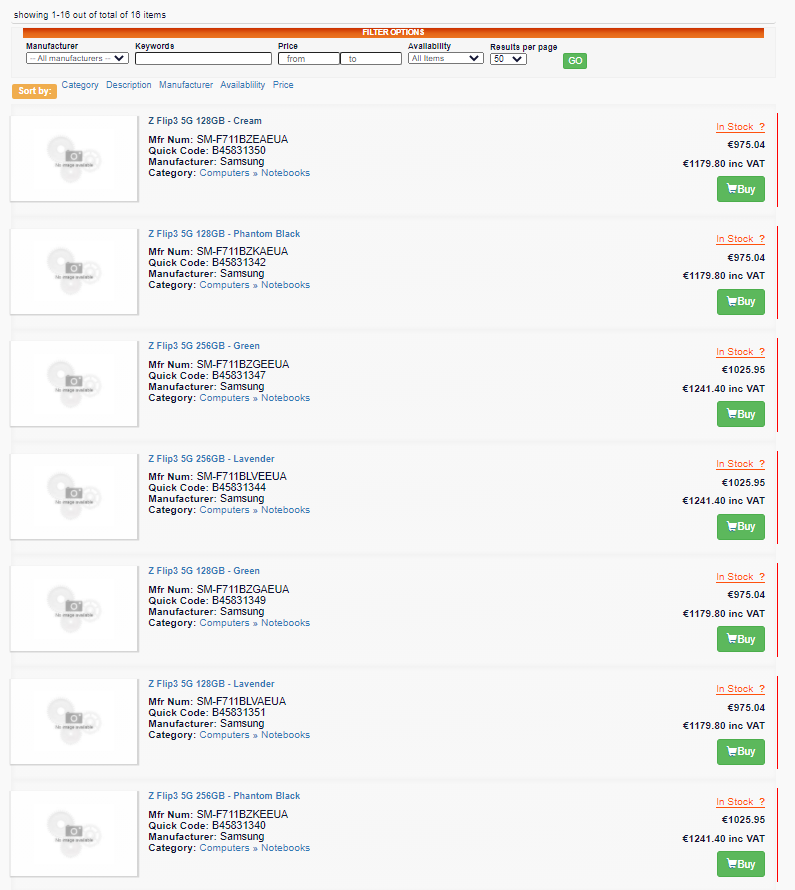Vertical web page layout displaying a product listing. 

The background transitions from light to medium gray at the top. In the upper left corner, in black text, it reads "Showing 1 to 16 out of a total of 16 items" above a thin gray line. Below this, there's an orange bar with "FILTER OPTIONS" in white uppercase text.

On the far left, the bold black headings include: Manufacturer, Keywords, Price, Availability, and Results Per Page. Under Manufacturer, a white drop-down box allows selection from "All Manufacturers." Similarly, there are white boxes for Keywords and Price, with "from" and "to" fields respectively. Availability is set to "All items" but can be altered via a clickable option. Results Per Page is set to 50, accompanied by a green "GO" button.

Further down, it says "Sort By" in orange. Clickable categories listed in blue are: Category, Description, Manufacturer, Availability, and Price. Below, a column of white boxes appears, each intended for product images but currently showing a camera icon with "No Image Available."

Next to each image placeholder, product titles appear in blue, followed by their descriptions, MFR numbers, quick codes, manufacturers, and categories in black text. Going across each entry, there's an "In Stock?" status in orange, prices in pounds, followed by prices including VAT. Each product has a green "BUY" button with a white shopping cart icon.